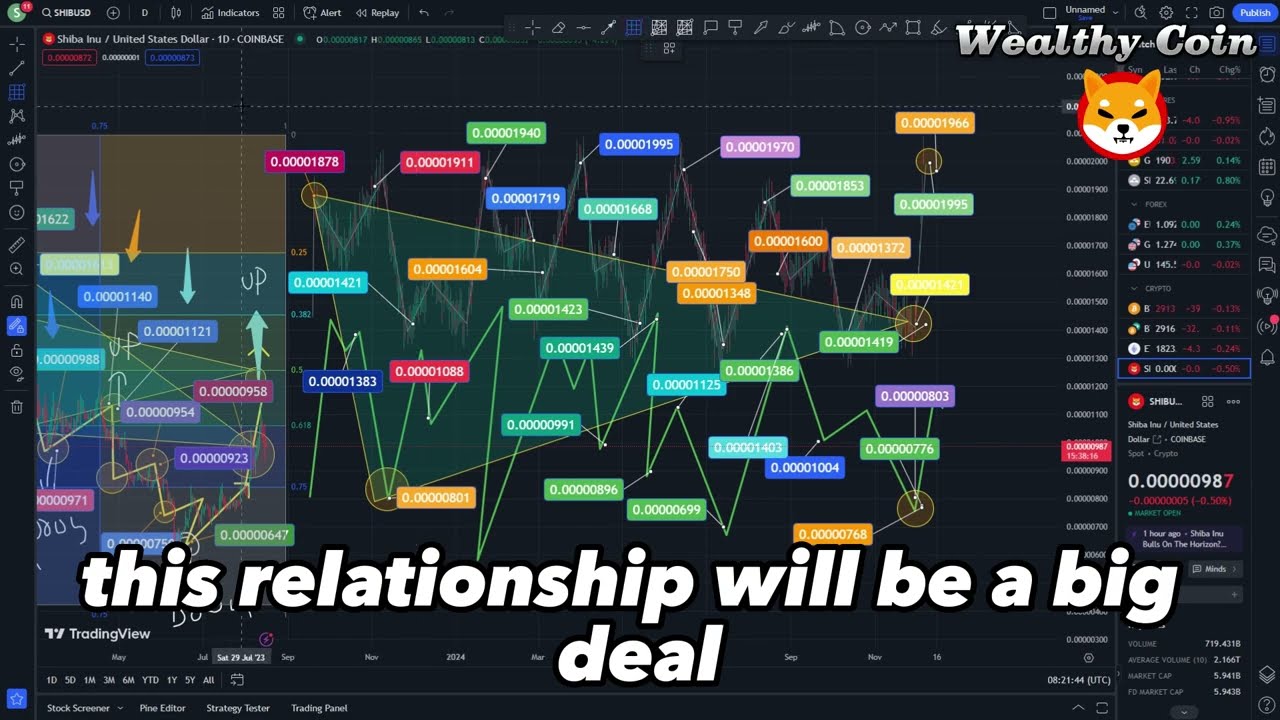The image is a screenshot of a computer application, specifically related to cryptocurrency trading. The background of the application is black, with a toolbar featuring various tools and icons located along the left-hand side and the top of the screen. At the upper right corner, there is a logo of Shiba Inu and a "wealthy coin" icon. The central part of the screen displays a chart of a financial asset, likely the Shiba Inu coin, featuring colorful graphical objects including a green zigzag line and a transparent green triangle. In the lower third of the screen, prominent text in white letters reads, "This relationship will be a big deal," which is divided into two lines, with the word "deal" on the second line. The screen contains a variety of tabs and columns with numerical data, adding detailed information relevant to cryptocurrency progression and trading activities.